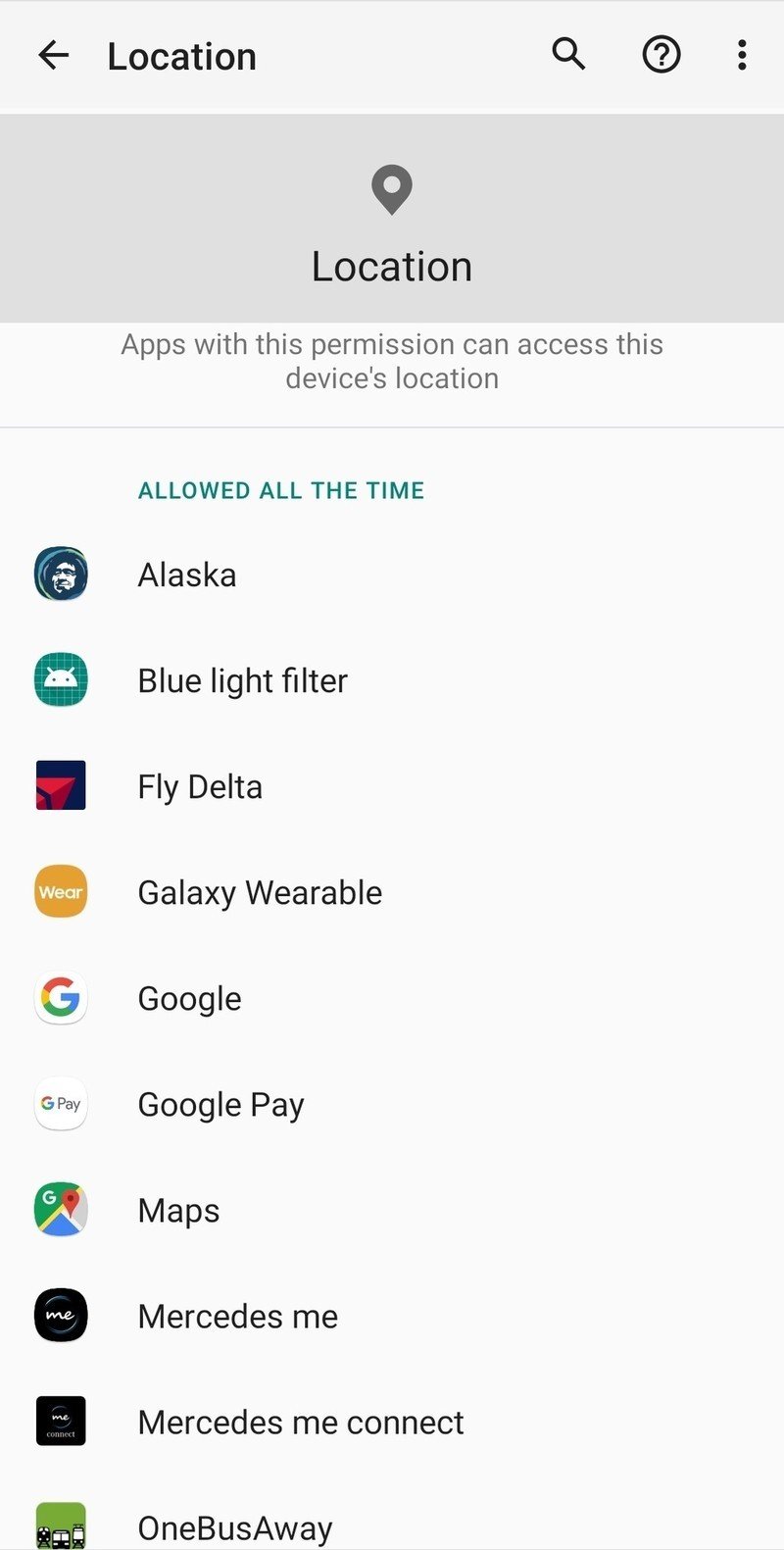This screenshot is from a cellular telephone operating system showcasing the "Location" settings page. The top section features a header on an off-white background. In the upper left corner, there is a black left-pointing arrow followed by the word "Location" in black, left-justified text. To the upper right, there are three icons: a black magnifying glass, a black circle with a question mark inside, and three vertical ellipses indicating the presence of a sub-menu that has not been activated.

Below the header, there is a thick gray bar approximately half an inch in height displaying the word "Location" in black text, accompanied by the familiar upside-down teardrop location icon. Beneath this bar, a small white banner with gray text informs the user that "Apps with this permission can access this device's location."

A thin, light-gray dividing line separates this banner from the menu items below. The menu lists various apps that have location permission, starting with "Allowed all the time" in aqua green text. Underneath this heading are various app names, each accompanied by their respective thumbnail icons, all left-justified. The listed apps include: 
- Alaska Airlines, represented by its icon
- Blue Light Filter with its specific icon
- Fly Delta with its recognizable thumbnail 
- Galaxy Wearable
- Google
- Google Play
- Maps (Google Maps)
- Mercedes me
- Mercedes me connect
- OneBusAway

Each app is aligned neatly, showcasing the different services that have permission to access the device's location.